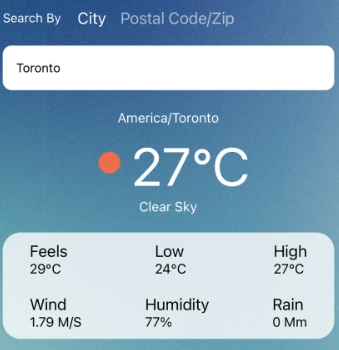**Screenshot of Regional Weather Guide for Toronto**

The image is a small screenshot featuring a weather or temperature guide with a blue background. At the top of the screenshot, there is a menu bar with options to "Search by" either "city" or "postal code/zip code." The city option is currently highlighted. In the search box below the menu bar, "Toronto" is entered, and the guide displays relevant weather information for the region.

The main weather display shows "America/Toronto" at the top, which identifies the regional context. Below this, large white characters prominently display the current temperature as "27°C," with a small red dot next to it, likely indicating a specific status or an alert. Directly below the temperature, the words "Clear Sky" describe the current weather condition.

Beneath this main weather summary, there is a separate, whitish rectangular window that provides additional detailed weather data in six fields:
1. **Overall Temperature:**
   - High: "27°C"
   - Low: "24°C"
   - Current: "29°C" (possible different or another current reading)
2. **Wind:**
   - Speed: "1.79 m/s" (interpreted as meters per second)
3. **Humidity:**
   - Percentage: "77%"
4. **Rainfall:**
   - Measure: "0 mm" indicating no rain

This detailed breakdown gives a comprehensive view of Toronto's current weather conditions, making it a useful tool for residents and visitors alike.